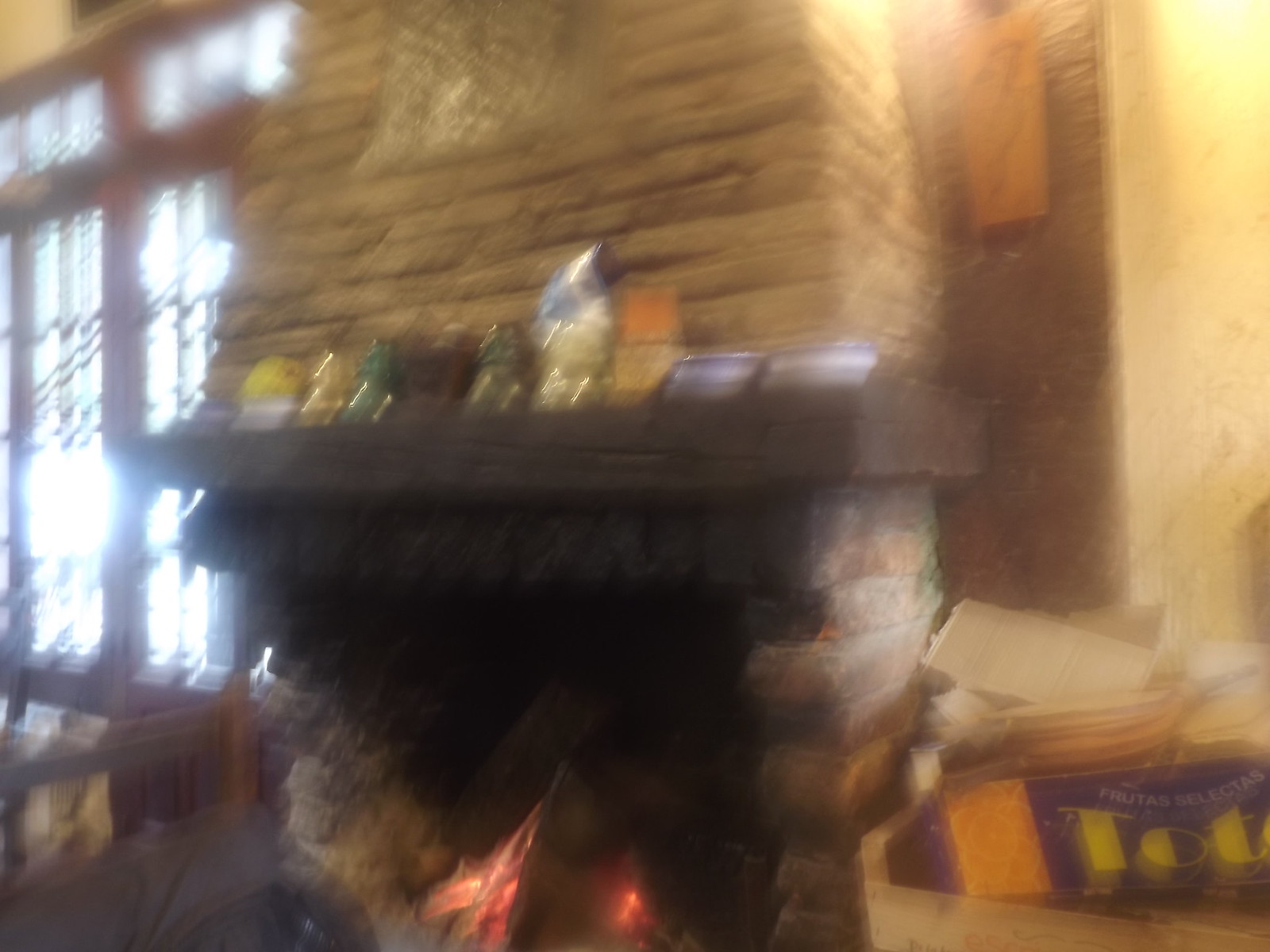The image captures a slightly blurry, indoor scene centered on a large, tan brick fireplace that exudes a sense of rustic warmth. The fireplace, reminiscent of one in a lodge or hotel, features an older, tall chimney reaching towards the ceiling, constructed of brown brick that matches the rest of the fireplace. The mantel, made of dark wood and echoing the coloration of surrounding trims, holds various decorative items including a blue and white bowl, a blue and white vase, and a short green and yellow vase, though the details are somewhat obscured by the blur. Orange and red flames are visible in the lower part of the fireplace, creating a cozy ambiance. Flanking the fireplace are tall windows with dark wood trim, featuring intricate scalloped designs. To the left of the fireplace sits a basket, possibly filled with books or magazines, adding to the inviting atmosphere. On the right, a small table or possibly a chair holds a cardboard box adorned with bubble print text reading "T.O.T." and some illegible white text, further contributing to the scene’s homey clutter. The cream-colored walls on both sides frame the fireplace, tying the composition together.